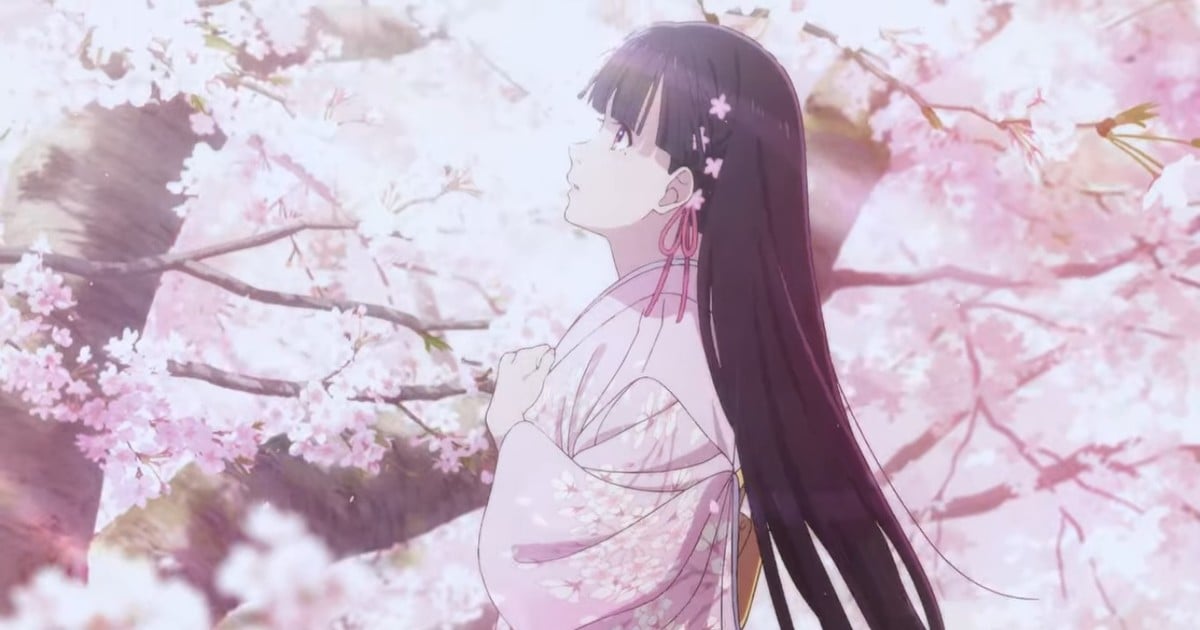The image depicts a Japanese anime-style drawing, potentially from a comic book, graphic novel, website, or video game. At the center is a young girl with long black hair adorned with bangs and pink flowers, and an additional small pink bowtie in her hair. She has wide-eyed wonderment, pale skin, and is wearing a traditional Japanese kimono robe featuring pale pink and white floral patterns. In the background, there are numerous branches of cherry blossoms (sakura) in full bloom, with delicate pink and white flowers on brown branches. The girl is the focal point of the image, standing out amidst the vibrant, floral background. There is no text visible in the picture, and the color palette includes predominantly black, white, various shades of pink, peach, and brown. A bright light seems to be shining on her from the top left, enhancing the enchanting and serene atmosphere.